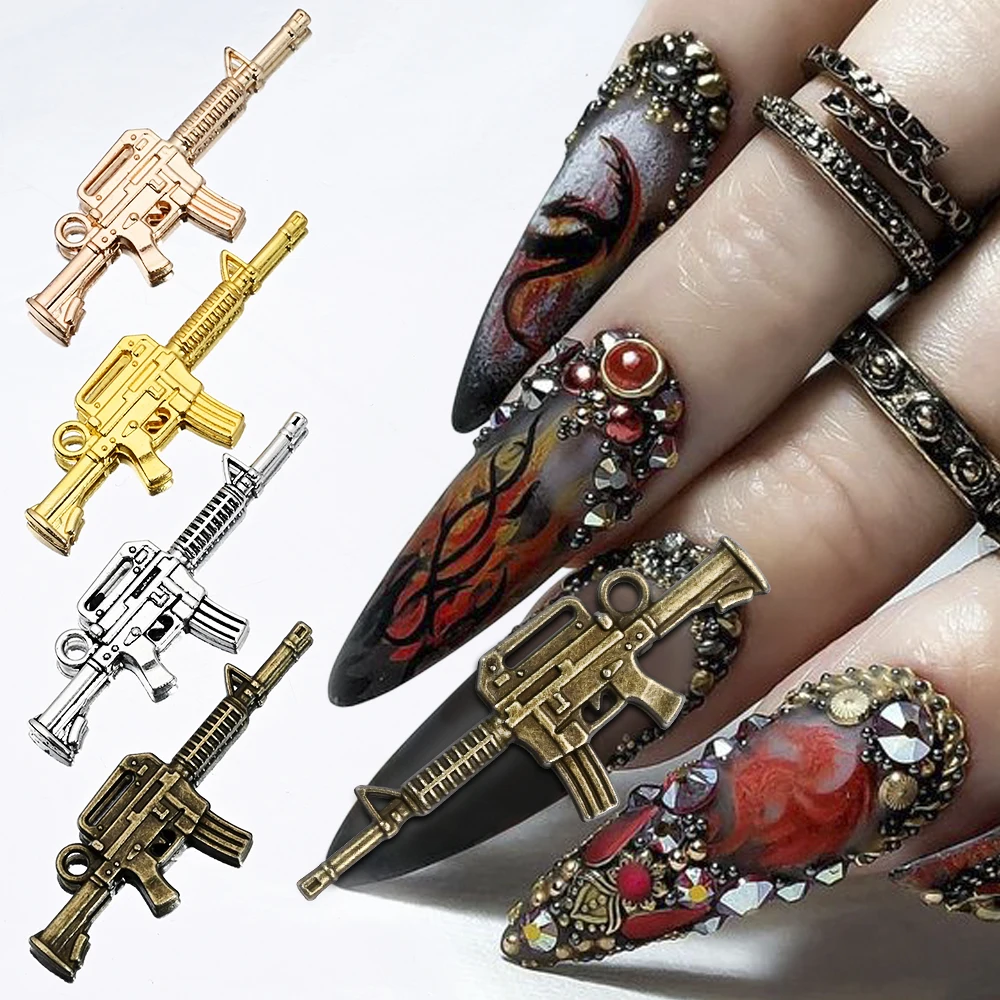In this photograph, an intricately manicured hand extends from the right side of the frame. Each finger showcases a unique and elaborate nail design, adorned with an array of decorative elements. The pinky finger features a sophisticated arrangement of gems and gold beads, while the ring finger boasts an abstract pattern with dark hues and pearl embellishments. The middle finger stands out with a miniature weathered gold M4-style Armalite rifle charm attached, adding a dramatic, bold touch. Small rings delicately adorn the tops of the middle and ring fingers, enhancing the overall opulence. The pointer finger at the bottom follows a vibrant theme, incorporating reds, transparent layers, and crystal accents.

To the left of the hand, four diminutive models of M16 rifles are displayed against a white background. Arranged in descending order, they are crafted from rose gold, yellow gold, silver or platinum, and a weathered gold—the latter matching the charm on the middle finger. Each miniature firearm features a small hoop, suggesting they can be worn as necklace pendants or bracelet charms. This impeccably detailed composition highlights the fusion of artistry and personal expression through avant-garde nail design.